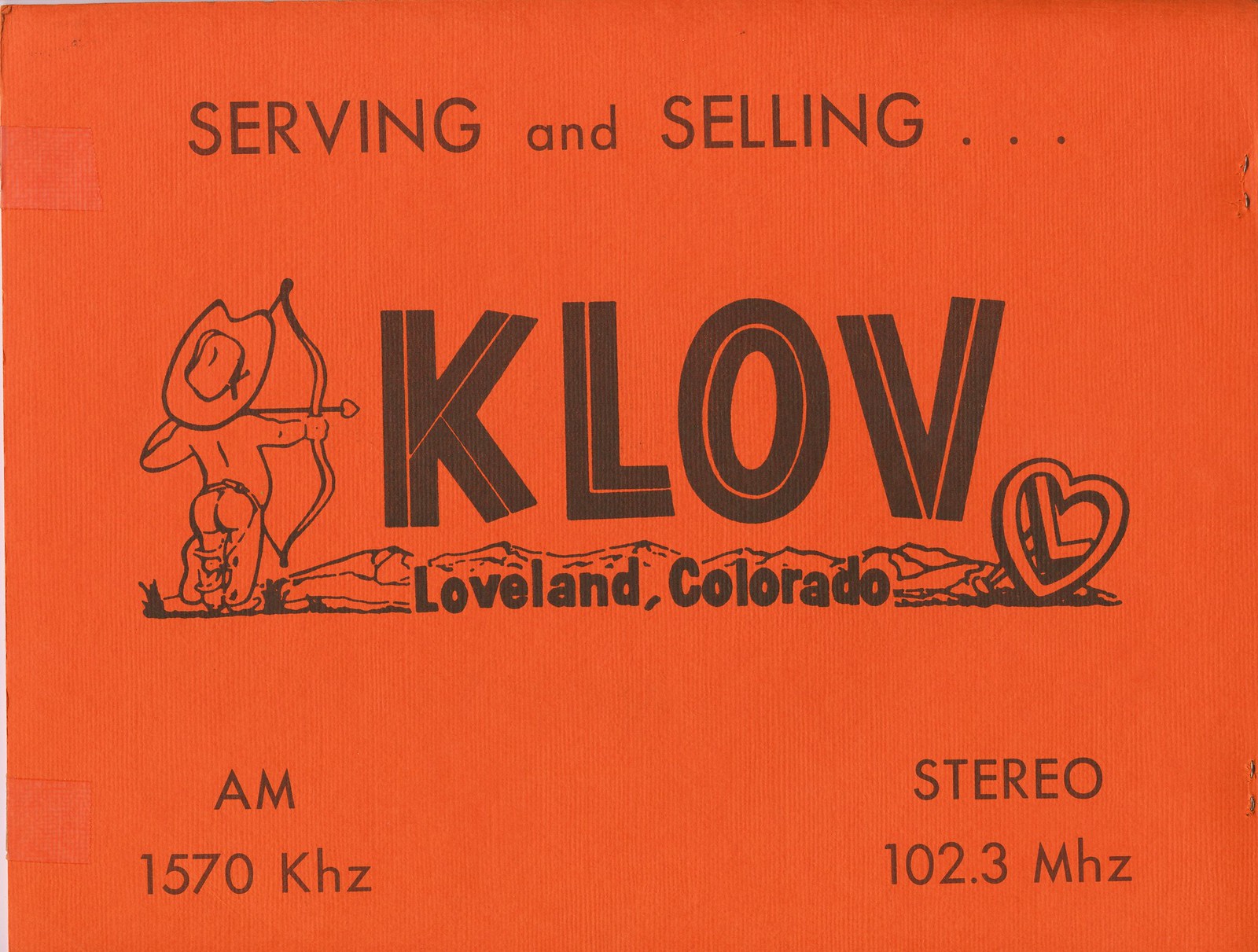This rectangular image appears to be an advertisement with a bright orange background and muted black print and images. Across the top, the text reads "Serving and Selling…" Below that, there's a striking illustration of a man dressed as a cowboy wearing chaps, a cowboy hat, and holding a drawn bow and arrow, positioned as if ready to shoot. The man is facing away, displaying his backside. To the far right, there's a heart with the letter "L" inside, accompanied by the text "KLOV," indicating "Loveland, Colorado." In the bottom left corner, the text reads "AM 1570 KHZ," while the bottom right corner displays "Stereo 102.3 MHZ." The overall appearance suggests a vintage advertisement for a radio station, possibly featuring slow rock or pop music.